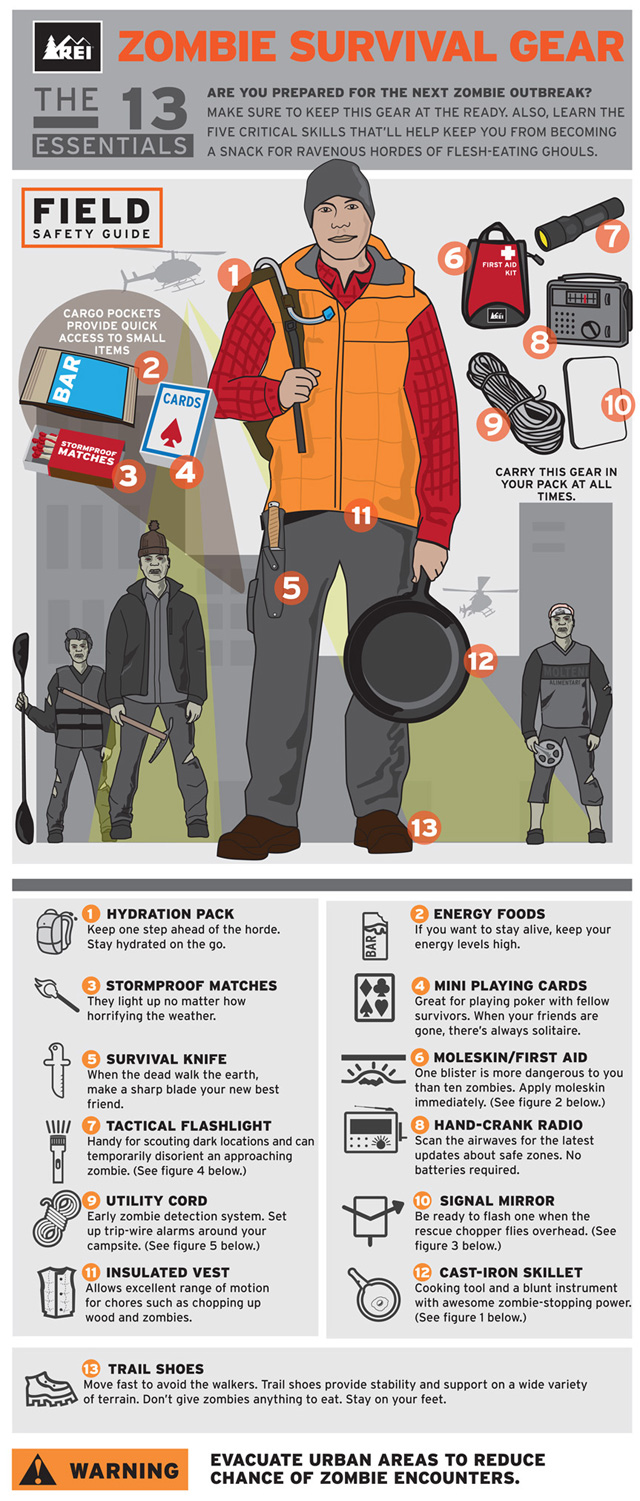The image is a detailed promotional poster for "Zombie Survival Gear," likely found in a magazine or on a webpage. Dominated by hues of orange, red, beige, black, green, gray, white, and blue, the poster prominently features a man decked out in survival attire, including an orange vest, red shirt, and grey pants. Surrounding him are various essential survival items labeled numerically from 1 to 13. Notable gear includes a hydration pack, storm-proof matches, survival knife, tactical flashlight, utility cord, insulated vest, trail shoes, energy foods, mini playing cards, moleskin first aid, hand-crank radio, signal mirror, and a cast-iron skillet. The top of the poster is inscribed in bold orange letters with "Zombie Survival Gear." Additional text alerts readers to prepare for the next zombie outbreak and highlights five critical survival skills. Flanking the man are images of menacing zombies, while detailed descriptions of each survival item appear below. The bottom section carries a stark warning to evacuate urban areas to reduce zombie encounters, emphasizing the crucial nature of having the right survival gear, possibly promoted by REI.